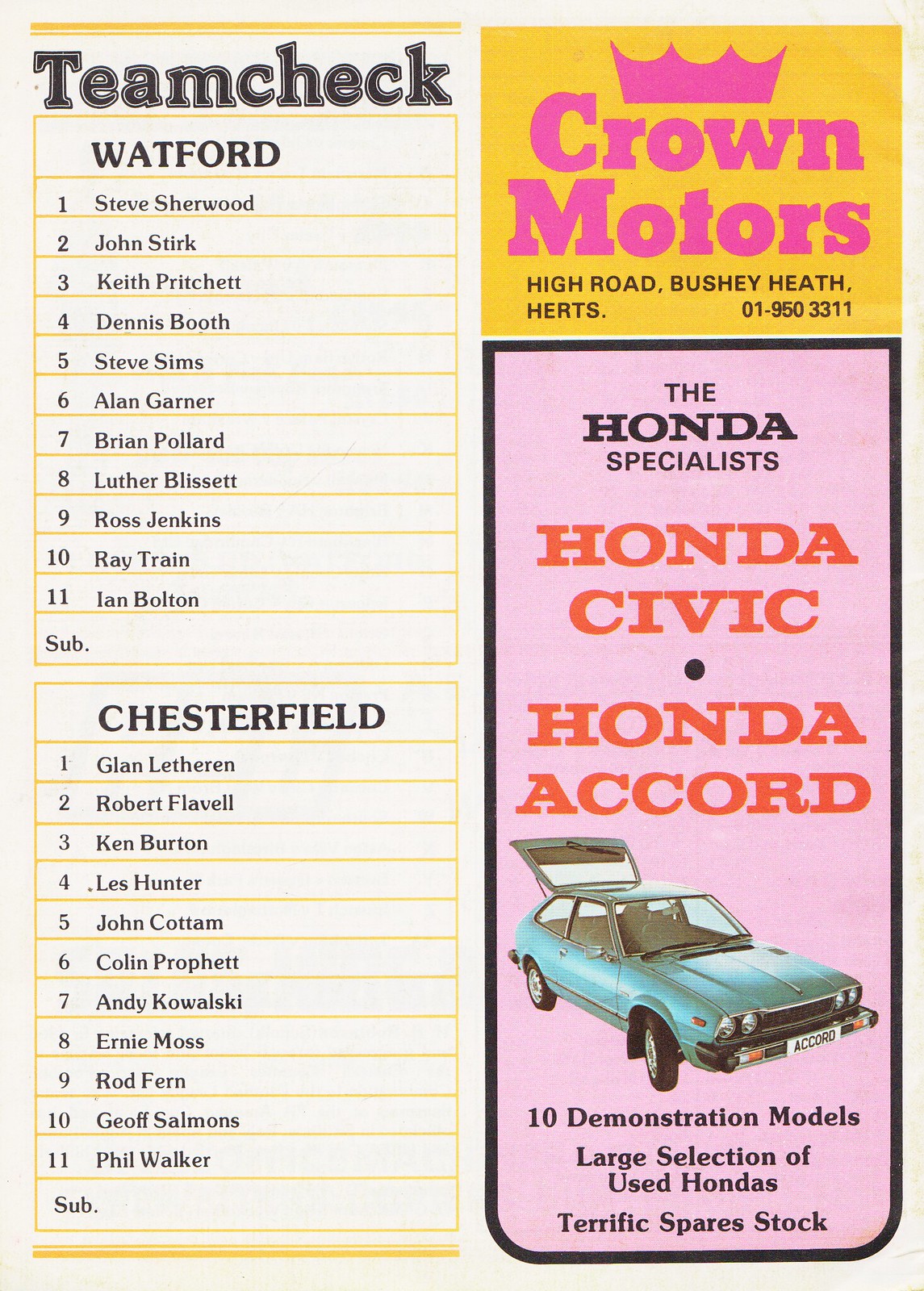This image is a detailed vintage print production from an old magazine, likely from the 70s, featuring a program page for a soccer match. It is composed of two columns on a cream-colored background. The left column is headed by "Team Check" in bold black lettering, listing the players' names and numbers from 1 through 11 for two teams: Watford and Chesterfield. The Watford team includes players like Steve Sherwood and Luther Blissett, while the Chesterfield team follows underneath. 

The right column features prominent advertisements. At the top, an ad for Crown Motors is displayed with a gold background and a pink logo, including a crown and the address "High Street, Bushy Heath, Hertz 01-950-3301" in black text beneath it. Below this, occupying about two-thirds of the column, is an advertisement for the Honda Specialists. It starts with "Honda Civic" and "Honda Accord" in red type on a pink background, followed by a photograph of a vintage blue Honda Civic hatchback. Additional information in black highlights "10 demonstration models, large selection of used Hondas, terrific spare stock."

The colors present in the image include shades of tan, yellow, pink, purple, orange, light blue, black, and gray. The setting and style suggest it is part of an insert or a program page from a car magazine with a nostalgic touch, emphasizing both soccer team details and car advertisements.